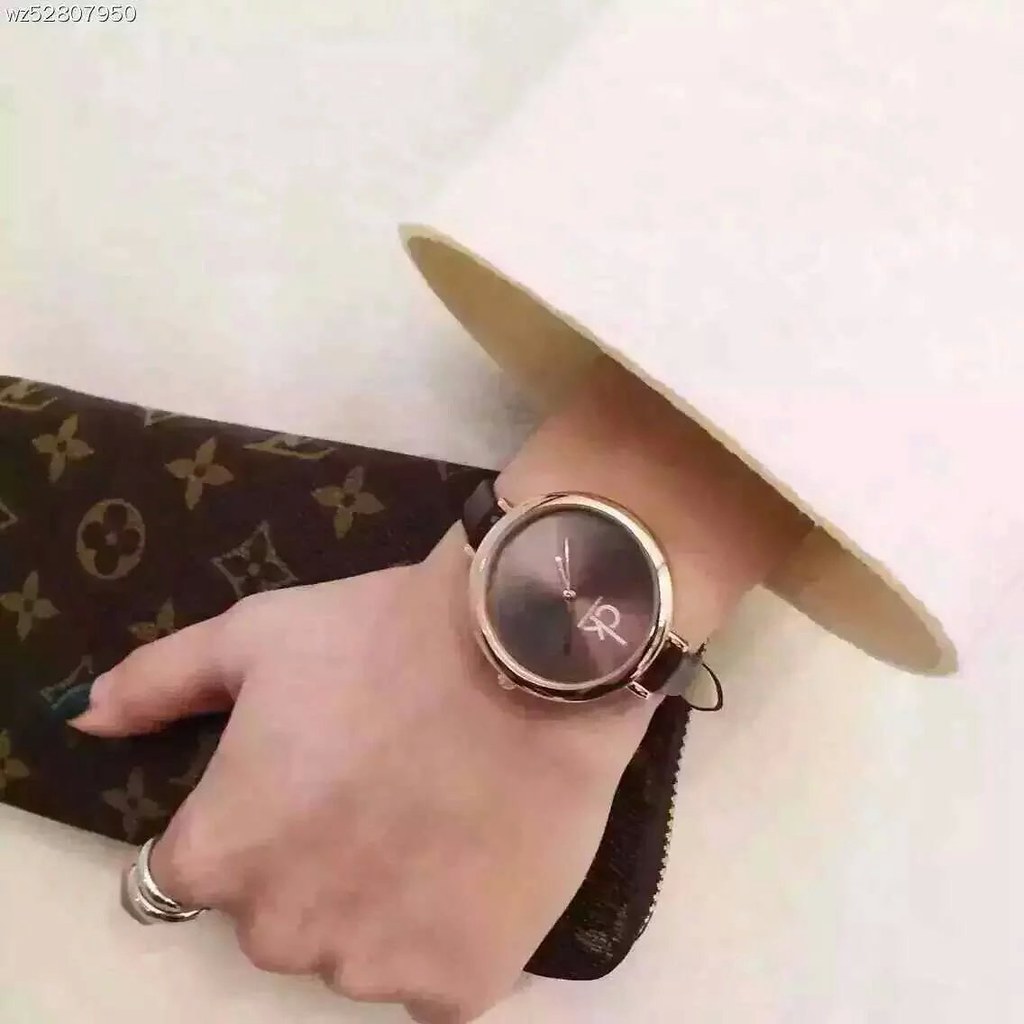The image showcases a close-up view of a woman's left arm and midsection, highlighting her elegant accessories. Adorning her left wrist is a sophisticated watch prominently featuring the initials 'CK'. Her arm is gracefully positioned such that the viewer's eye is drawn from her elbow down to her waist, stopping just above her belly button. In her left hand, she elegantly holds a luxurious Louis Vuitton handbag, easily identifiable by its signature pattern of interlocking 'L's and 'V's. The handbag itself is a rich brown color, accentuated by subtle lighter brown shading, enhancing its classic and timeless appeal.